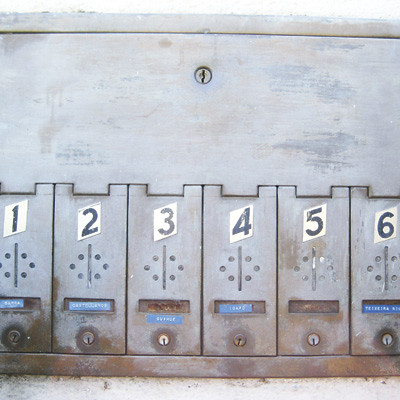This photograph depicts a row of old-fashioned mailboxes, likely situated in an apartment building. The mailboxes are made of a grayish metal, tinged with hues of light brown, suggesting wear and age. The focal point showcases a wide, drawer-like door extending the full width of the image; this upper compartment features a small keyhole for unlocking, presumptively used by the mail carrier to distribute the mail.

Below the main door are six smaller rectangular mail slots, each assigned a unique function. At the top of each slot, a white sticker with black numbers from one to six identifies the individual boxes. Just below these numbers, there is a peculiar design: a straight vertical line bordered on either side by three dots arranged in a triangular pattern.

Further down, each box has a designated space for name tags. These name tags are created using a label maker, forming embossed letters on little blue strips. The horizontal indentation where the name tags are affixed reinforces the nostalgic charm. At the very bottom of each slot is another keyhole, enabling residents to retrieve their mail. The overall appearance of the mailboxes, with their slightly tarnished and aged look, evokes a sense of vintage functionality.